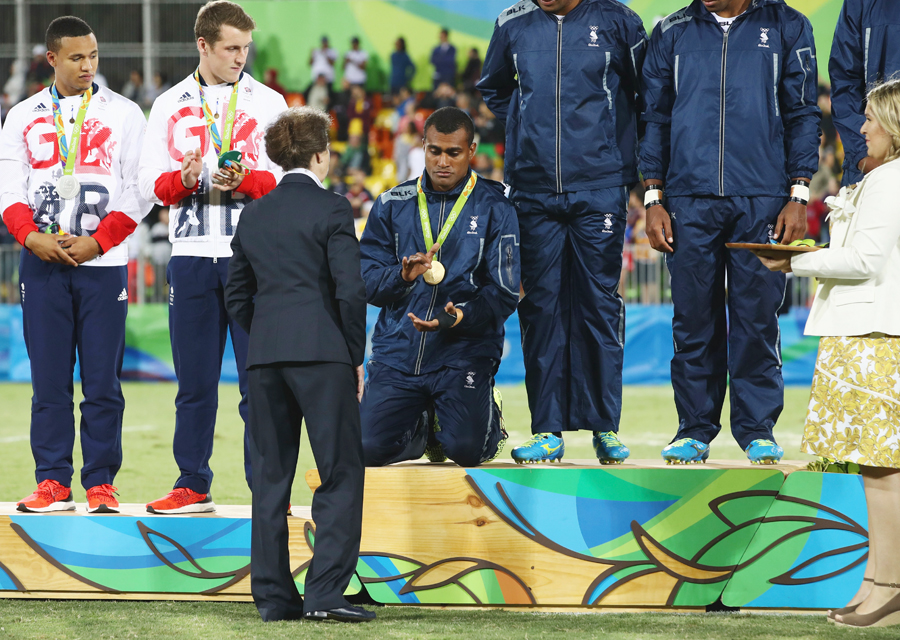This photograph captures a detailed moment during a sports award ceremony featuring a line of six male athletes, all dressed in track suits. The scene is set on a raised stage. The two men on the left are dressed in blue sweatpants, white jackets adorned with red and blue lettering, and red sneakers. Each of them proudly displays a medal around their neck. The four athletes to the right wear matching blue track suits and teal Nike sneakers, with the central figure in this group kneeling down, apparently mid-clap, sporting a green-ribboned medal around his neck. To the kneeling man's left, two men also exhibit medals and look on, one clapping. To the far right, a woman in a yellowish print skirt and white jacket holds a tray that seemingly contains more medals, their green ribbons visible. Another woman, dressed in a suit with her hair up, stands with her back to the camera, facing the kneeling man, likely having just presented him with his medal. The photograph captures the moment of recognition and celebration among the athletes and presenters.